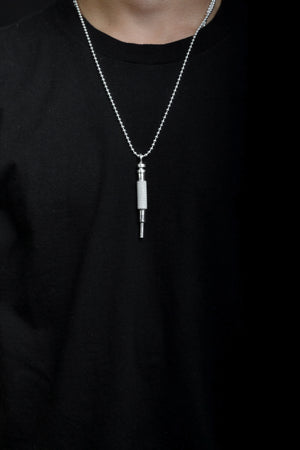In the image, we see the chest and a small portion of the neck of a fair-complexioned man wearing a plain black t-shirt that has some wrinkles. The focus of the picture is a silver chain necklace around his neck. The chain appears slightly uneven on one side, and it holds a pendant shaped like an audio jack plug, resembling the tip of an amplifier cable, which is also silver and white. The overall scene suggests the possible presentation of a product, as the head and other body parts of the individual are not visible, clearly highlighting the necklace and its unique pendant.